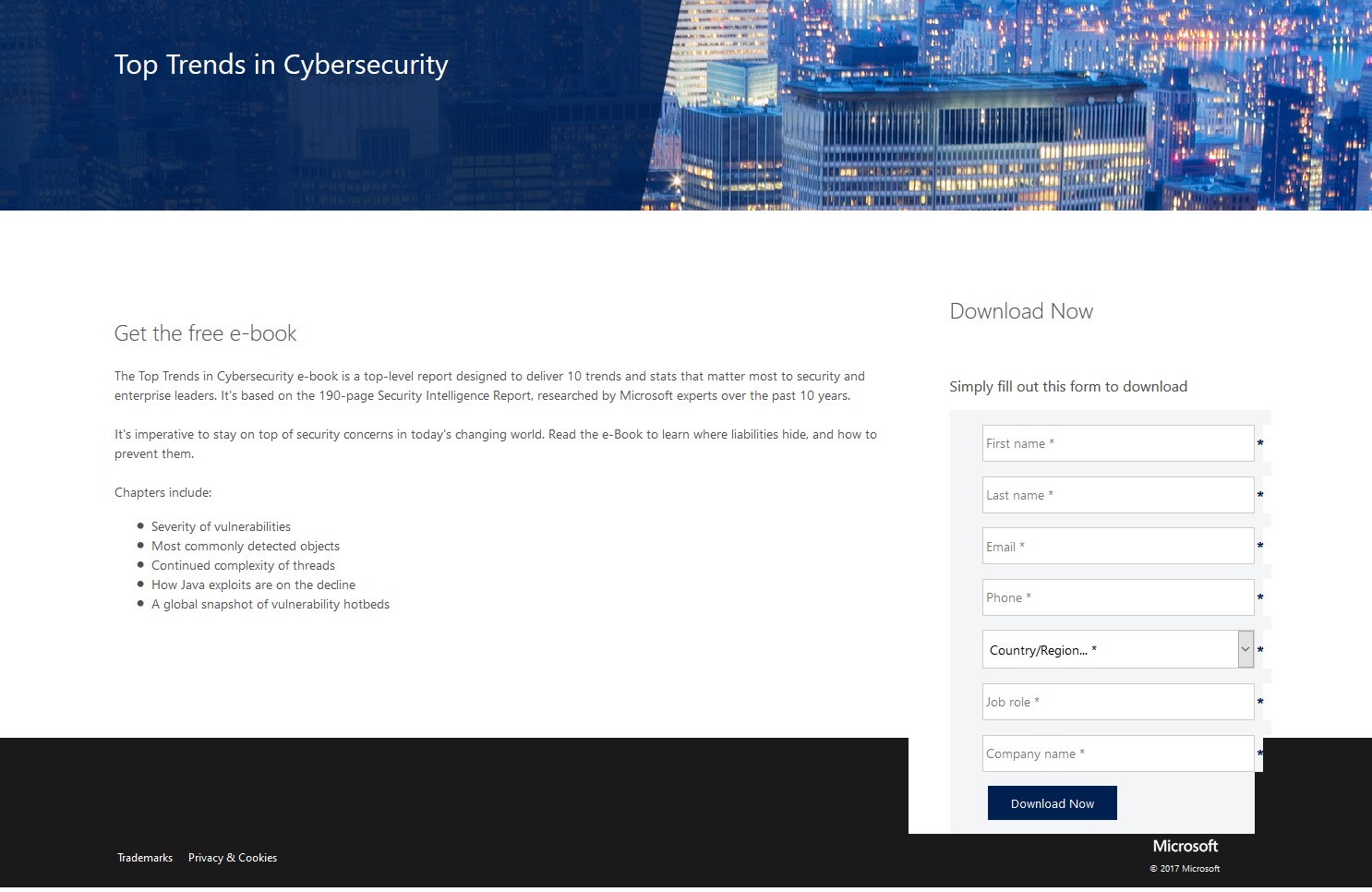An aerial night view of a bustling cityscape serves as the dynamic background for the Top Trends in Cybersecurity website banner, prominently positioned at the upper left-hand corner in sleek white font. The city's myriad buildings are illuminated, creating a vibrant tapestry of lights against the dark sky. Below the banner, a call-to-action section invites visitors to "Get the Free E-book." This e-book, a comprehensive top-level report, outlines the 10 most critical trends and statistics in cybersecurity, crucial for both security and enterprise leaders. Drawing from a meticulously researched 190-page security intelligence report by Microsoft experts, accumulated over the past decade, it aims to equip readers with essential insights into potential liabilities and preventive strategies in the ever-evolving landscape of cybersecurity.